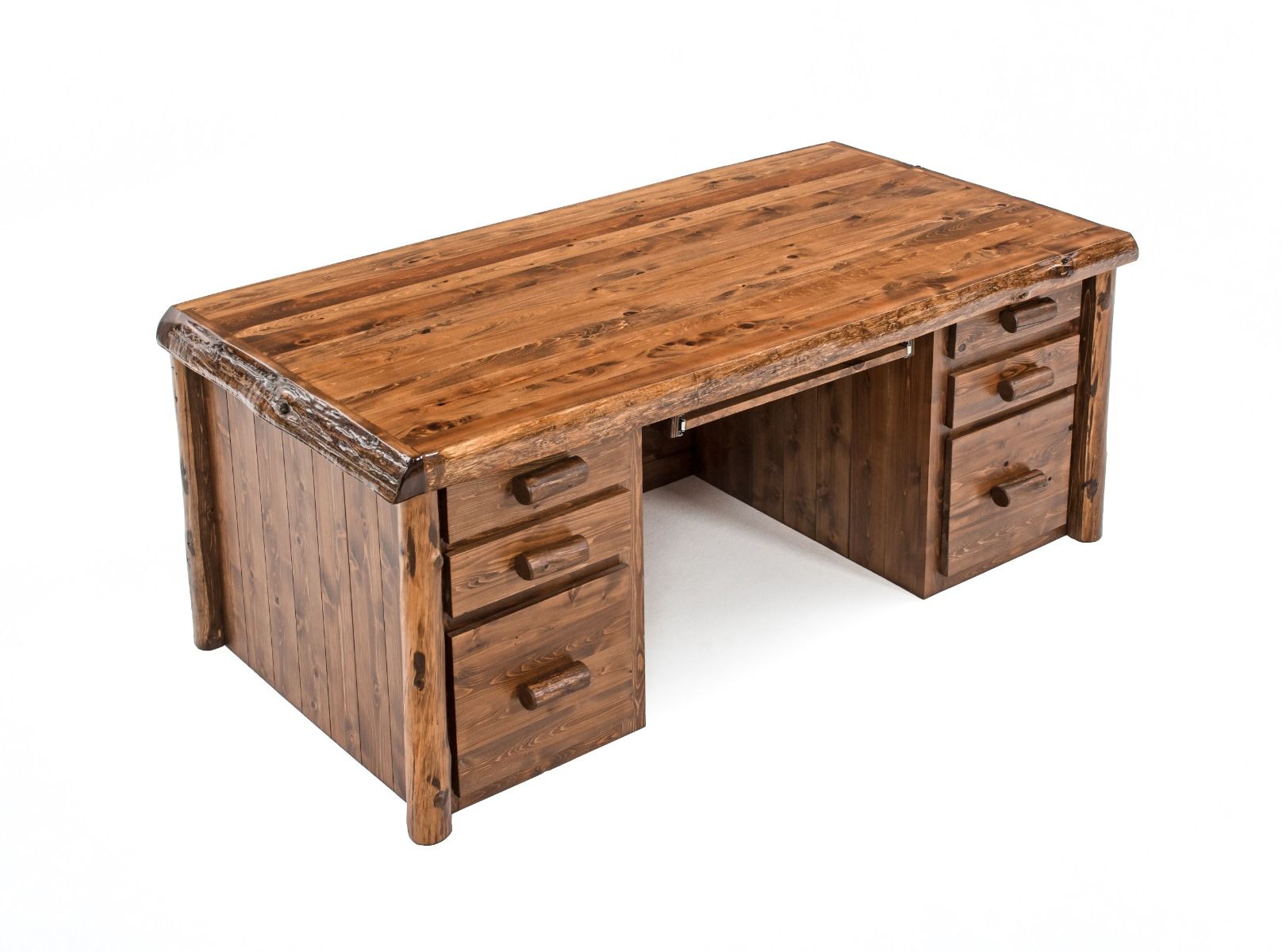The image features a large, robust, rustic wooden office desk, showcased against a bright, plain white background. The desk is very chunky and appears quite heavy, constructed entirely from solid wood with a stained finish that ranges from a dark mahogany to walnut color, exhibiting rich variations in wood tones. The desk has an old-fashioned, handcrafted charm, reminiscent of a wood cabin-turned-desk. 

It features spacious, symmetrical storage with a set of three drawers on each side of the seating area—two smaller drawers stacked above a larger one on both the left and right sides, akin to the size of file cabinet drawers. The drawers are adorned with wooden handles and are surrounded by vertical lines on the side panels, suggesting they were built from different wood pieces. Additionally, there's a pull-out tray situated underneath the main desk surface, potentially useful as a keyboard tray. 

The edges of the desk are unique, formed by live wood with natural bark, adding to its rustic appeal. The corners of the desk are supported by thick, rounded wooden legs resembling stripped branches or narrow tree trunks. This photo captures the entire structure of the desk, including the leg space and underneath area, reinforcing its sturdy, woodland-style character.